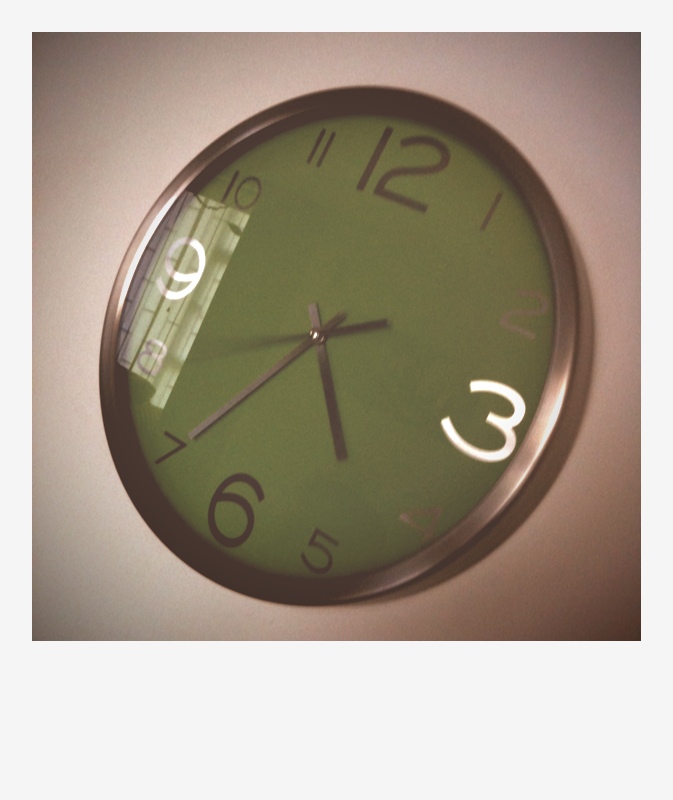This is a detailed close-up photograph of a wall clock set against a beige background, presumably the wall it hangs on. The clock itself is a shade of dark green, possibly appearing lighter due to minimal shadowing in the image. Its design is modern and minimalist, featuring large numerals for 12, 3, 6, and 9, while the remaining numerals are smaller in comparison. This analog clock is covered by a plastic shield that reflects light, revealing the faint image of window panes, suggesting a nearby light source. Notably, the numerals at 9 and 3 appear white, compared to the black numerals for 12, 6, and most of the others, excluding the 2, 4, and 8, which display in a dark gray or silver hue. The overall aesthetic is simple and functional, with an intriguing play of reflections adding complexity to the image.